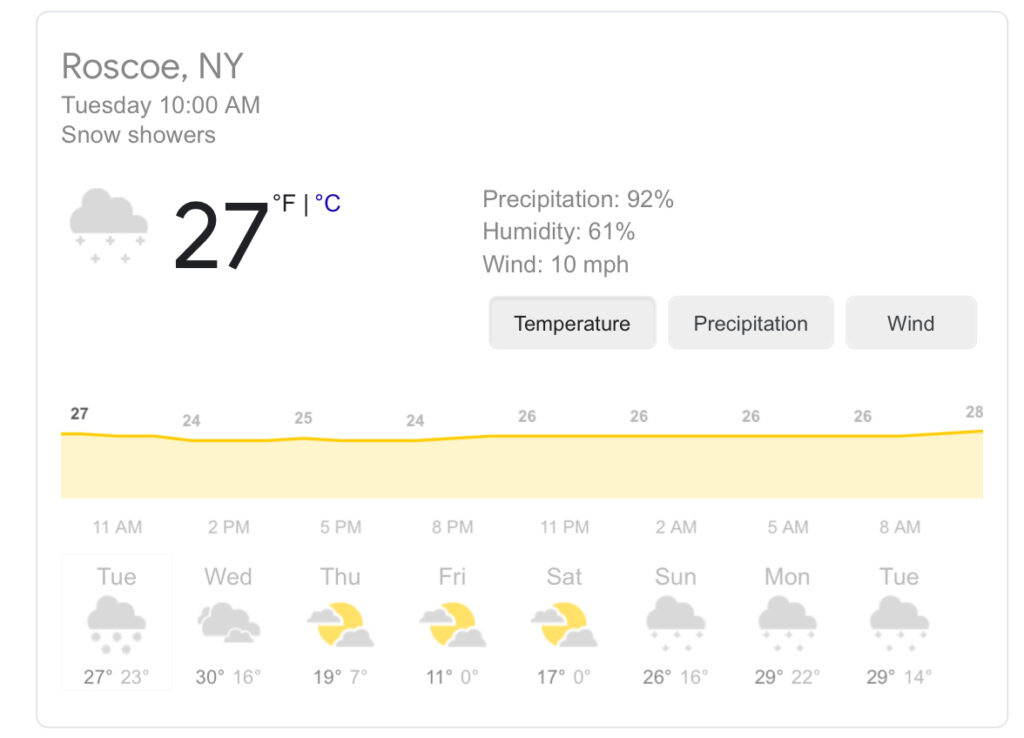Screenshot of an eight-day weather forecast for Roscoe, New York displayed in the upper left corner. The current weather at 10:00 a.m. on Tuesday shows snow showers with a temperature of 27°F. The weather icon depicts clouds and snowflakes, with a 92% chance of precipitation, 61% humidity, and winds blowing at 10 mph. 

In the center of the screen, there are buttons for "Temp," "Precipitation," and "Wind." A color-coded horizontal graph spans the duration from Tuesday through the following Tuesday, illustrating temperature fluctuations with a jagged line. The temperatures range from 27°F to 28°F, marked at different times of day from 11 a.m. to 8 a.m.

Each day from Tuesday to next Tuesday shows symbols indicating varied weather conditions, including partial sunshine and clouds, with the high and low temperatures displayed underneath each day's icon. The forecast includes maximum and minimum temperatures for each day, providing a comprehensive weather outlook. The image has a white background, giving the diagram a clean and basic appearance.